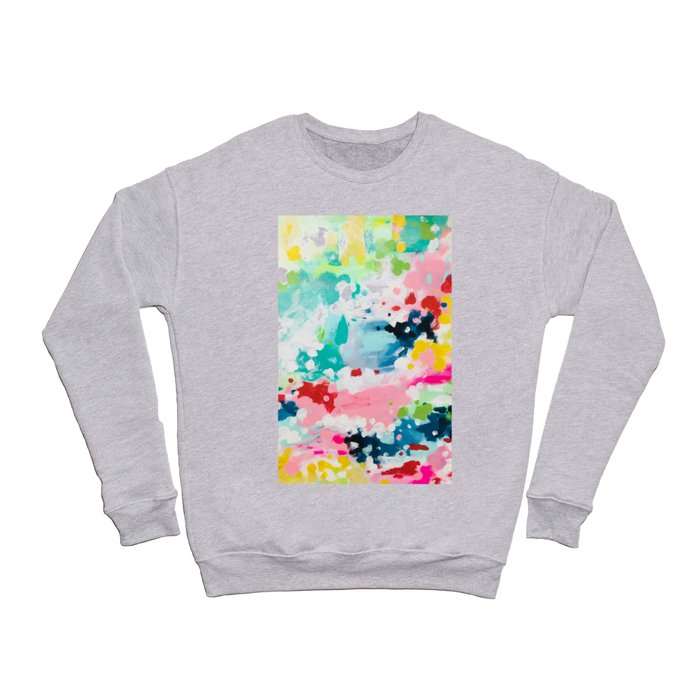This photo features a light gray, lightweight sweatshirt with long sleeves. The sweatshirt has ribbed cuffs, a ribbed band at the bottom, and a scoop neckline. At the center of the sweatshirt's front is a prominent rectangular print displaying an abstract pattern of colorful splotches. This modern art-inspired design includes a diverse palette of colors such as yellows, greens, teals, pinks, reds, and various shades of blue, all set against a white or possibly transparent background. There are no tags or text visible on the shirt. The vibrant pattern appears to be a decal that covers a significant portion of the sweatshirt's front, adding a bold and artistic touch to the overall garment.